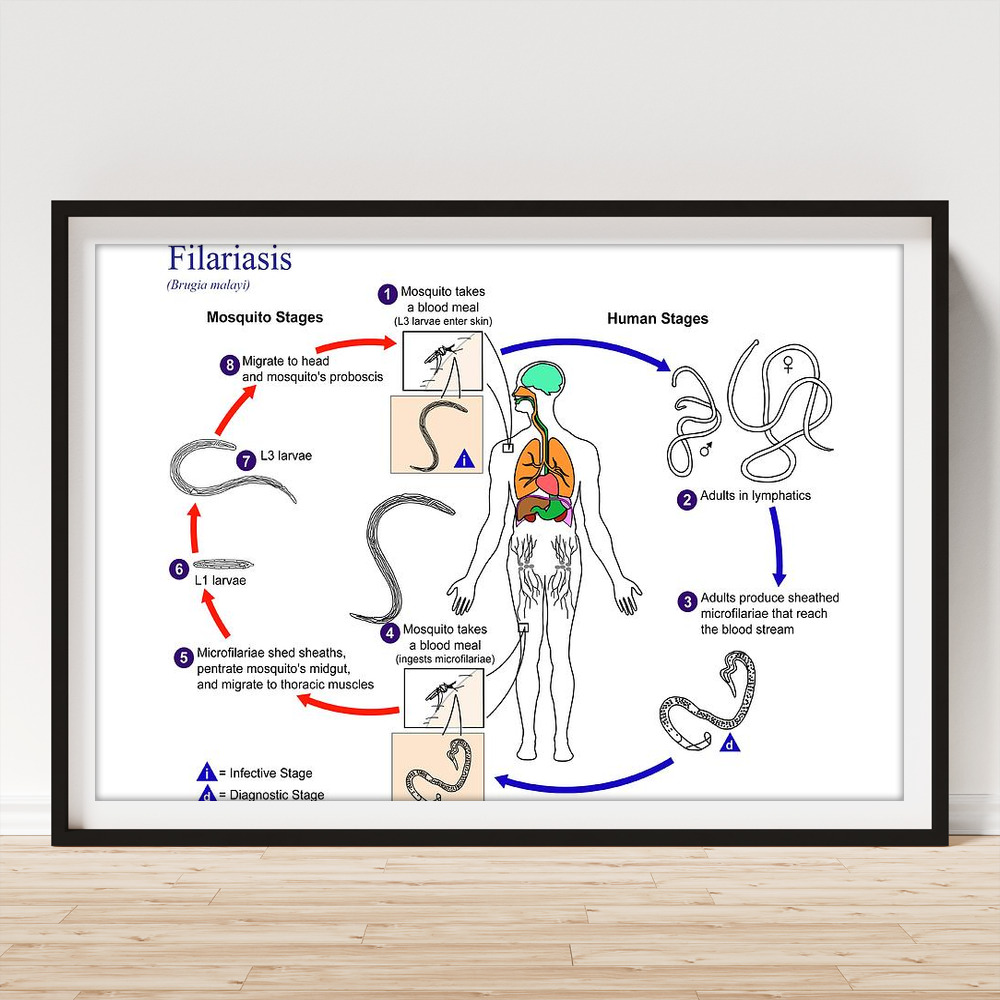The illustration, framed against a light gray wall with a wooden platform in front, serves as an educational medical chart detailing the life cycle of filariasis, caused by Brugia malayi. The image features a central human figure, displaying internal organs in various colors: the brain in green, the lungs in orange, the heart in red, the liver in brown, and the stomach in green, among others. The chart is bordered by a gray frame and contains a series of eight labeled stages, depicting both human and mosquito phases of the parasite's life cycle.

In the top left corner, the word "FILARIASIS" is prominently displayed. The cycle starts with a drawing of a mosquito taking a blood meal (Stage 1), marked with an exclamation signifying the infective stage. The illustration follows the parasite's journey through the human body, where the larvae enter the skin, mature into adults in the lymphatic system, and produce sheathed microfilariae (Stage 3). These microfilariae reach the bloodstream, indicated by a diagnostic mark (Stage D).

The cycle continues with another mosquito bite, where the mosquito ingests the microfilariae (Stage 4). Inside the mosquito, the microfilariae shed their sheaths, penetrate the midgut, and migrate to the thoracic muscles (Stage 5). The larvae develop through stages L1 and L3 (Stages 6 and 7) and finally migrate to the mosquito's head and proboscis (Stage 8), completing the cycle.

Red arrows connect the mosquito stages, while blue arrows guide through the human stages. The illustration contains several technical details and markings to emphasize both the infective and diagnostic stages, enhancing its educational value.